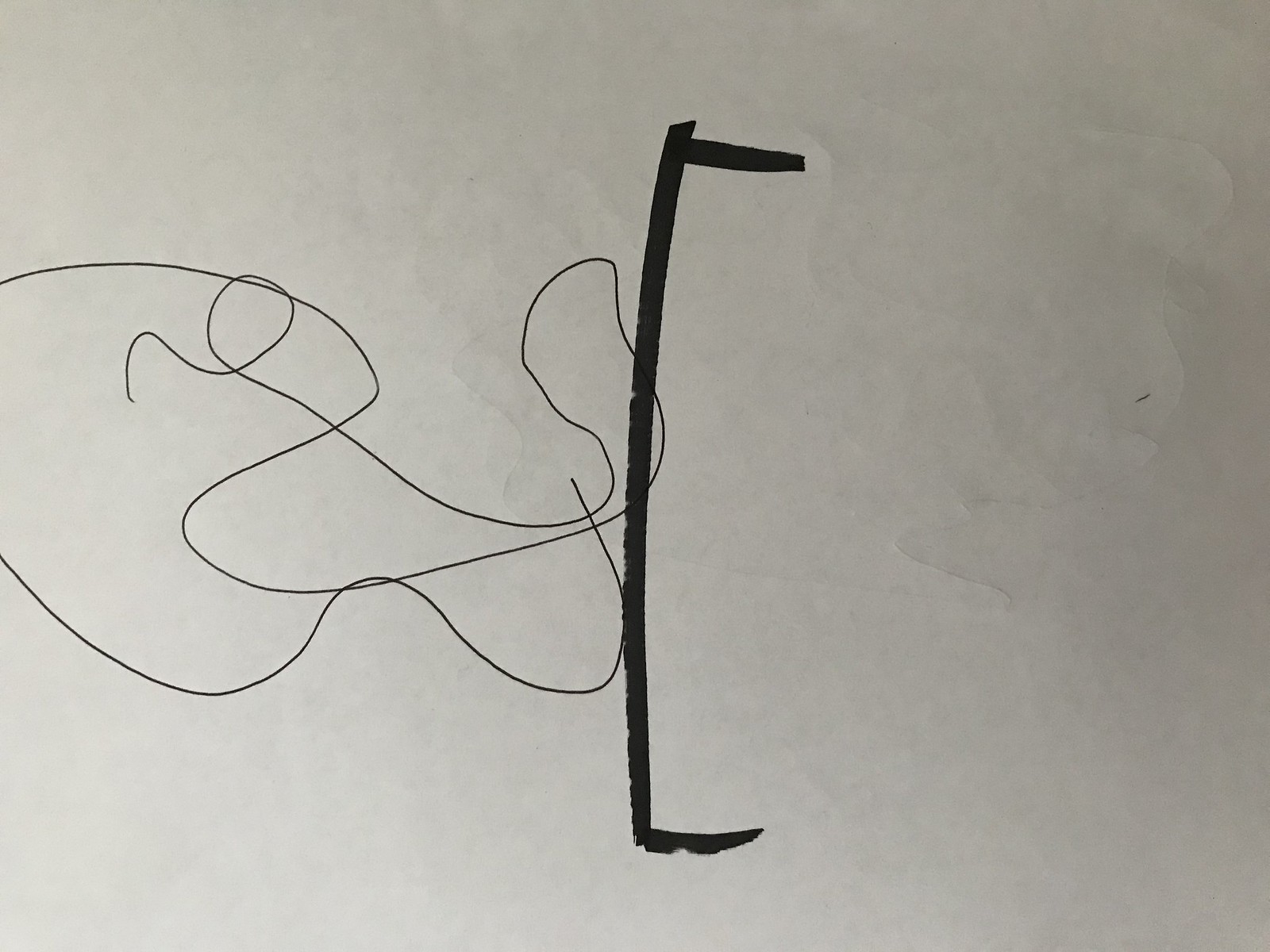The image appears to be either a drawing on a piece of paper or a whiteboard. The right half of the composition is blank, while the focal points are centered around the middle and the left sections. Dominating the center is a thick black line resembling the shape of a staple, with the ends that would typically bend inward pointing towards the right. This line, though not technically a staple, is drawn in a bold and substantial manner. 

Towards the left of the image, there is a white, swirly line that loops over itself multiple times, reminiscent of a long strand of black hair placed on a surface, perhaps to mimic the way one might stick hair on a shower wall to prevent it from going down the drain. This intricate line appears continuous and intersects the black, staple-like design at several points.

The overall impression is that of a photocopied or drawn scene, potentially featuring an abstract interaction between the staple-like figure and the swirling hair-like line. The precise rationale behind such a depiction remains ambiguous.